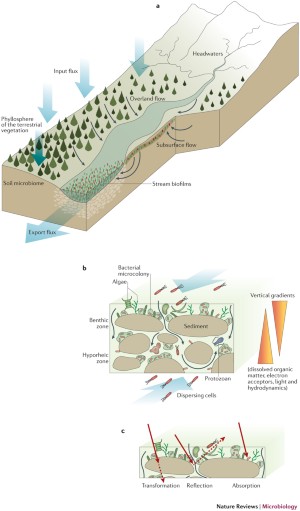The image appears to be an educational illustration taken from a science textbook, focusing on geological and hydrological concepts. At the top, there's a detailed 3D cutaway diagram of a landscape, showing a forest on the left, a river flowing downhill from a mountain on the right, and the underground path of water. The water's flow is indicated with numerous arrows, demonstrating how it travels through and erodes the land. This upper section also features several small text labels, which are too tiny to read. Below this, a middle image shows various parts of the land, split into sections to highlight different geological features and water interactions. At the bottom of the illustration, there's another diagram of the land in a beige-tan color, with two red, spiky triangles—one pointing up and one pointing down—emphasizing specific processes occurring in the land. The entire illustration has a white background, ensuring that the viewer's focus remains on the described geological and hydrological features.